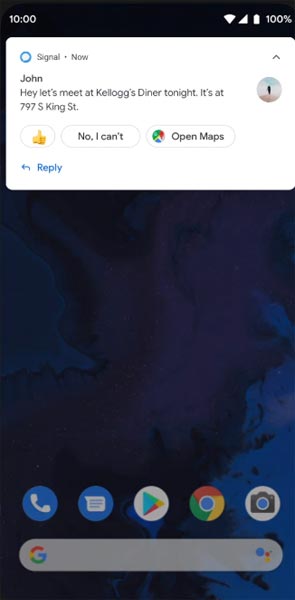A vibrant image captured on a smartphone screen, featuring a rich, artistically-blended background of deep bluish-purple and black hues. At the top of the screen, the status bar displays the time as 10:00, with full Wi-Fi connectivity, a solid white triangular signal icon, and a battery icon at 100%. Overlaying this colorful background is a white notification rectangle containing a message. The message reads, "John, hey, let's meet at Kellogg's Diner tonight. It's at 797 South King Street." Beside the message, on the right, is a small circular profile picture frame, depicted as a black silhouette. Below the message are three actionable buttons: a thumbs-up icon on the left, a middle button labeled "No, I can't," and on the far right, a small map icon with the text "Open maps." Additionally, there is a blue arrow pointing to the left accompanied by the word "Reply."